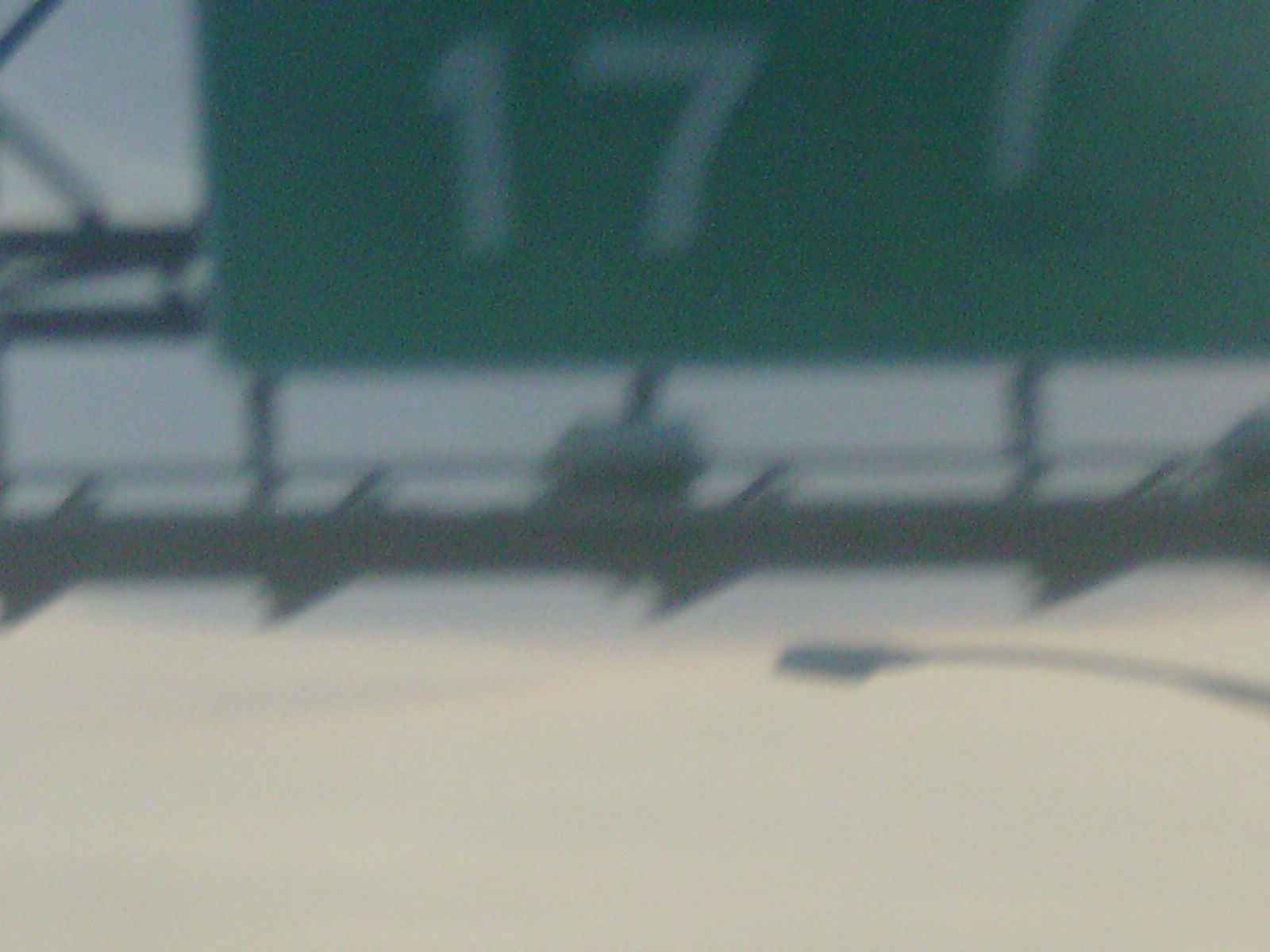The image captures a highway sign from a bottom-up perspective, showcasing the underside of a metal structure, likely an overpass or bridge, that supports the sign. The structure and attached sign create a silhouetted effect against a backdrop of a yellowish-gray sky merging into a darker blue hue. The green highway sign, blurred and pixelated due to the zoomed-in nature of the photograph, prominently features the white numbers "17." Although mostly obscured, there appears to be a curving arrow or line partially visible on the sign. Directly below, extending from the metal beams, is a streetlight that is silhouetted and unlit. The metal infrastructure is distinctly segmented, with visible joints, and there is a subtle hint of an underpass walkway below it.